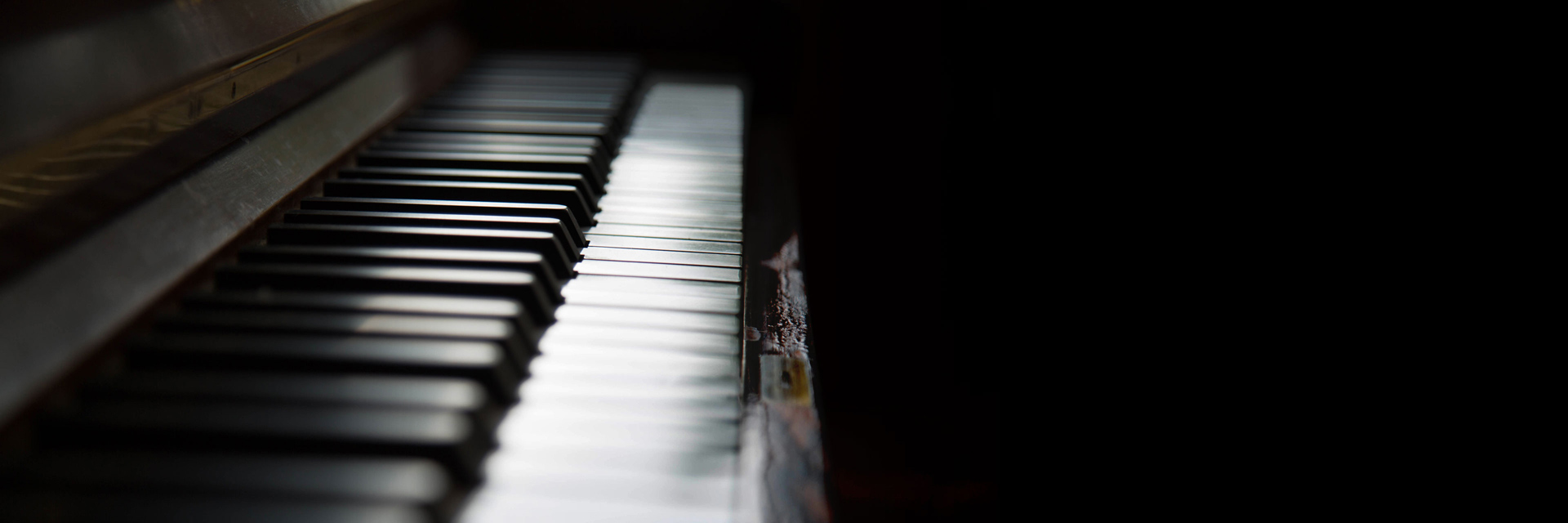This image is a striking close-up of a piano keyboard captured from a unique perspective. The photograph, horizontal in nature, emphasizes the pristine black background that sharply contrasts with the gleaming keys. The viewer's angle suggests looking down from the left side of the piano, giving a sense of descending into the keys. The white and black keys extend from the left corner of the image up towards the right, gradually shrinking in size due to the camera's perspective. Light shimmers off the glossy black keys, enhancing the artistic and tasteful presentation intended by the photographer. The upper portion of the piano is visible, along with the wooden cover typically used when the piano is not in use. Notably, there's an indistinct white and brownish object to the right center of the keyboard, although its purpose is unclear. Heavy gray shadows appear on the front of the keys, hinting at a targeted light source that accentuates the shiny surface, enhancing the overall elegant effect of the photograph.